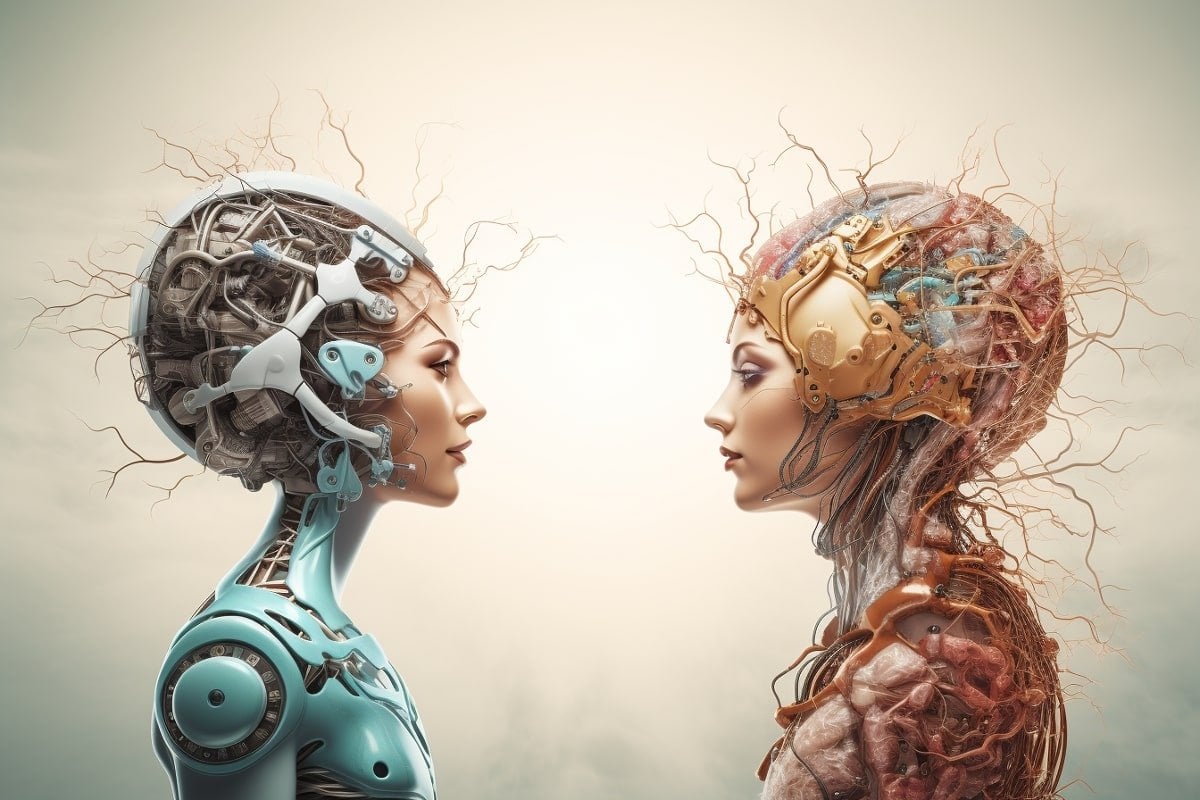This digital artwork showcases two female androids, portrayed in profile facing each other against a gradient beige-to-gray background. The android on the left has a body composed of blue metal with intricate gears at the shoulders and visible wires and computerized connectors inside exposed sections of her body and skull. Her very human-like face, with fair skin and light brown eyebrows, contrasts sharply with her mechanical form. The android on the right has a body made of red metal parts, which are heavily laden with wires extending from various sections, including the skull region. She, too, displays a highly realistic female human face with lighter blonde eyebrows. Both androids' heads reveal complex internals resembling computer network equipment, with wires sprouting almost like hair. Their aesthetic evokes a blend of mechanical precision and human beauty, set against a subtle, softly transitioning background.